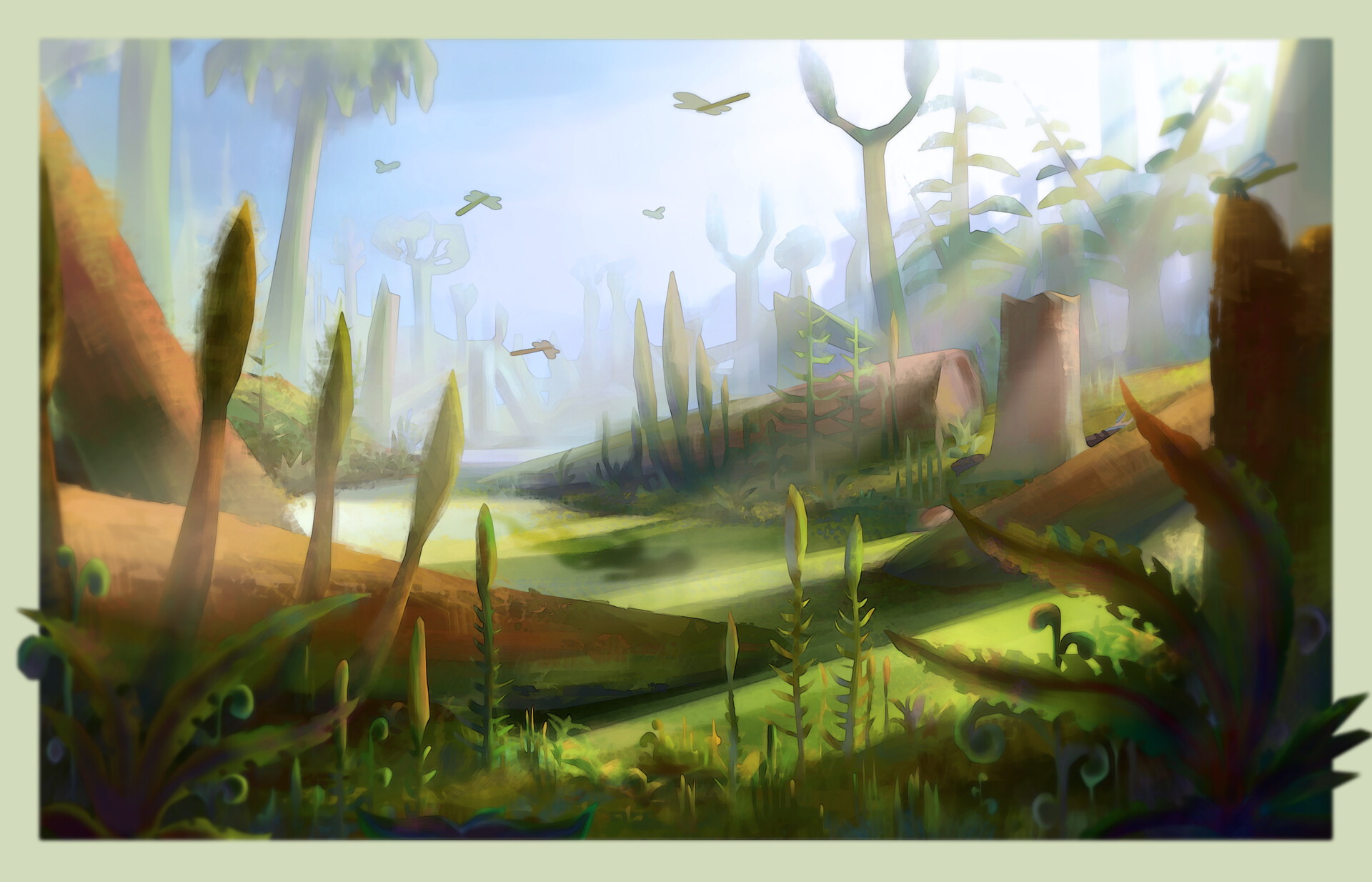This detailed artwork, possibly AI-generated, depicts a serene, hazy landscape reminiscent of the Zelda video game style. The entire scene is framed by a light green border, giving it an ethereal feel. Sunlight streams down from the upper right, casting a gentle illumination across the blue sky and the lush greenery below. The foreground features an array of plants and ferns, with some extending slightly beyond the borders of the image. Scattered throughout the scene are fallen tree trunks, interspersed with towering, wispy trees that add to the mystical atmosphere. Various insects, including rounded dragonflies, float in the air, enhancing the sense of a living, breathing ecosystem. The overall muted and blurred appearance of the image creates a dreamy, almost otherworldly ambiance.